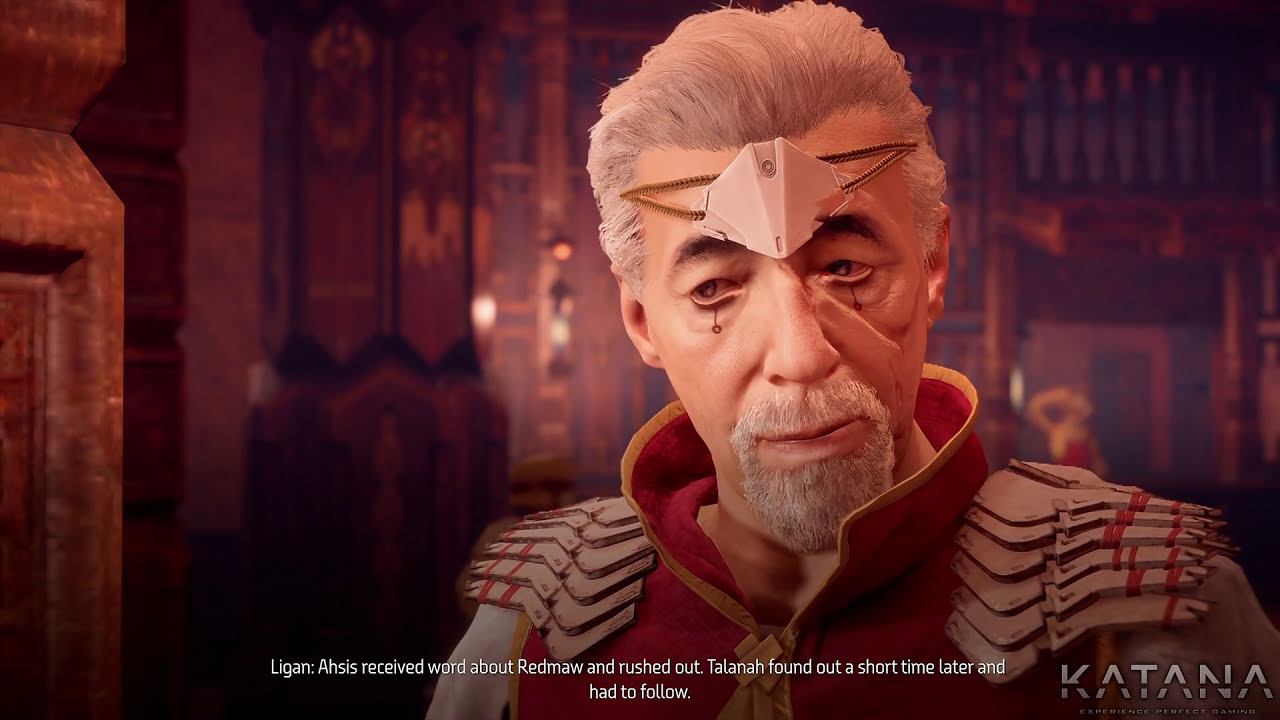The image depicts a detailed scene from what appears to be a lifelike video game or possibly an automated animated movie, with the main focal point being an older man, likely around 50 or 60 years old. He is a white man with wavy grey hair, a grey mustache, and a goatee. He is wearing a tan and red outfit that has an almost armor-like quality, adorned with echelons on the corners of his garments. On his head, he wears a headband with what appears to be a small plaster or crown-like accessory above his eyebrows. The outfit is further detailed with a collar that transitions from yellow to orange. 

The background is slightly out of focus but suggests a rich, intricate setting reminiscent of a library or a castle's interior, with visible wooden walls, windows, and possibly castle-like architectural features. The environment is lit softly, adding depth to the scene without drawing attention from the central character. 

On the bottom part of the image, white text reads: "Lygon, Ossus received word about Redmo and rushed out, Talonov found out a short time later and had to follow." In the bottom right corner, the word "KATANA" is prominently displayed, potentially indicating the name of the movie or the producer. The main colors featured in the scene include red, tan, and brown, contributing to a warm and somewhat ancient atmosphere.